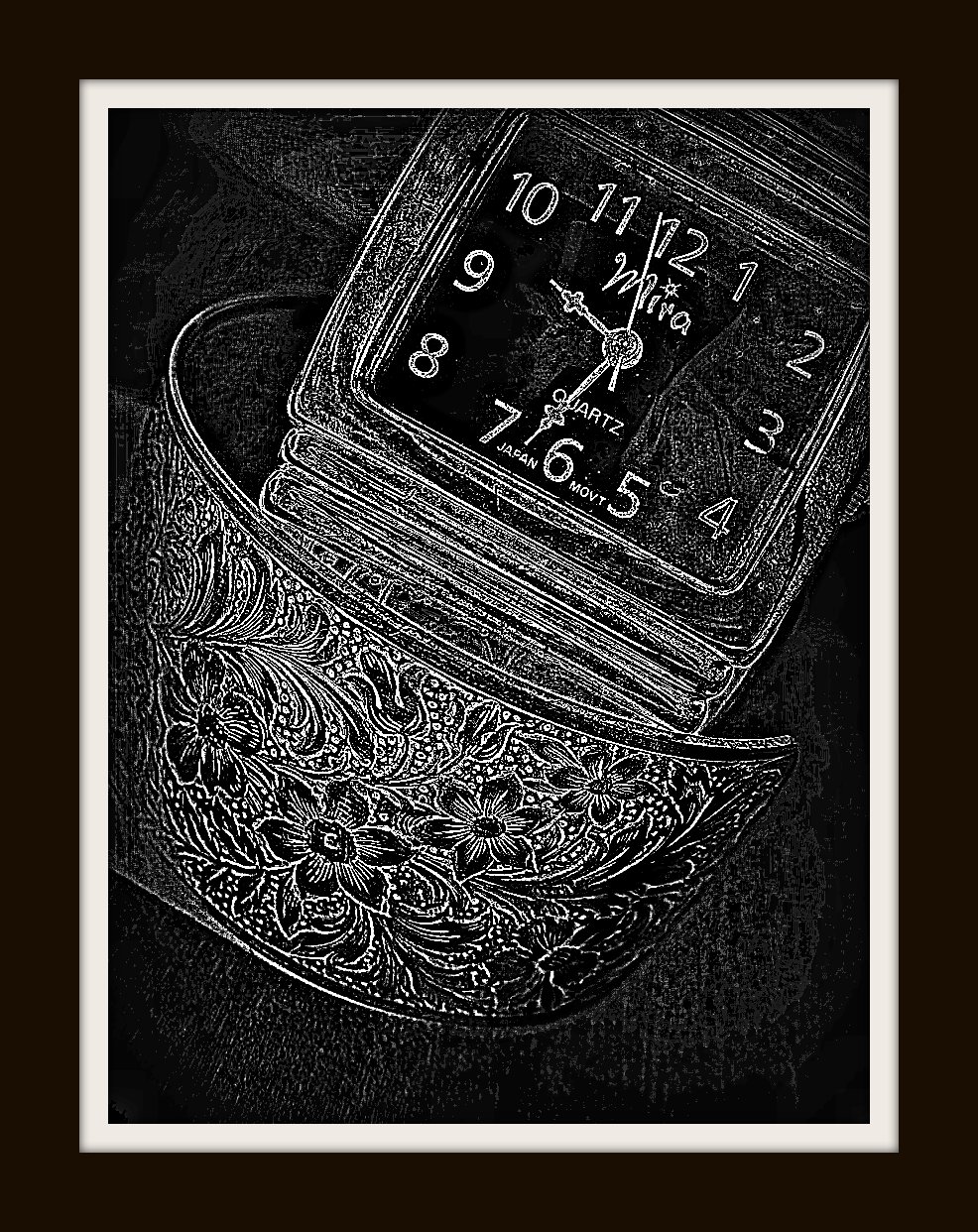This black and white image features a striking and intricate composition set against a pitch-black background. At the center, a white square frame encloses a further expanse of black, creating a layered and dimensional effect. The primary focal point within the frame is a detailed etching or line drawing of a watch, prominently displayed against the black backdrop.

The watch showcases a square face with hour markers numbered from 1 to 12. The white hands of the watch indicate that the time is between 6 and 7 o’clock, while the smaller hand points between 9 and 10. A seconds hand is almost perfectly aligned with the 12 o'clock marker. Above the watch hands, there is an unreadable logo inscribed in white, and below the hands, the word "quartz" is discernibly written.

Part of the watch's metallic bracelet extends from the frame, adorned with a delicate floral design, which seems to entwine around the bottom section of the bracelet. This floral element could either be an artistic decoration or a separate object placed in the scene. The composition rests on a surface that has subtle white grain patterns running through it, which are barely visible against the predominantly black background. The image masterfully blends elements of timekeeping with artful details, creating a captivating visual narrative.